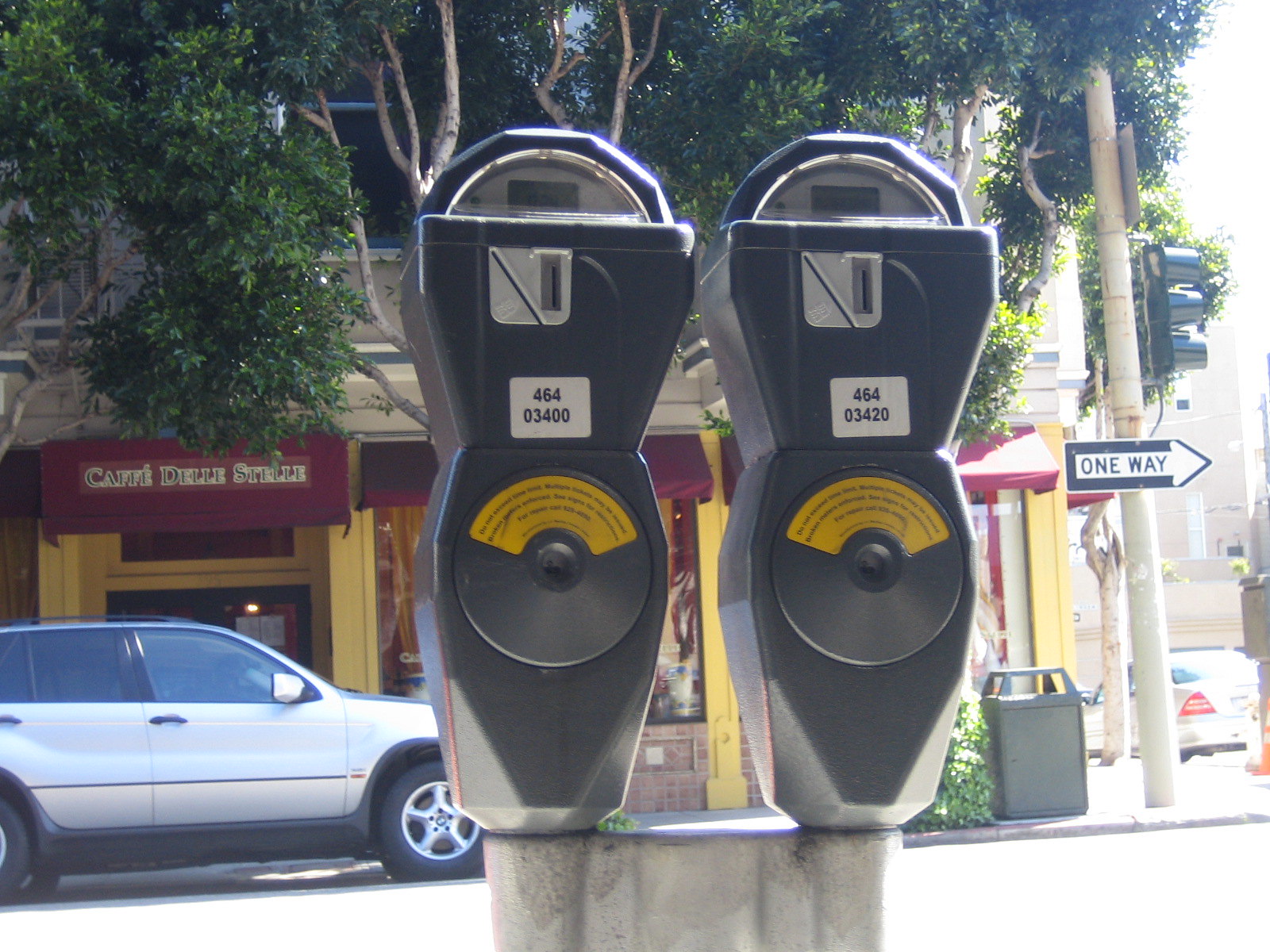The photograph features a close-up view of two black parking meters situated side-by-side on a city street during the middle of the day. Each meter sports a sticker with the numbers 46403400 and 46403420, respectively, and includes a yellow section containing small text, positioned near what resembles a knob for adjustments. The design of the meters is traditional, rounded at the top with visible dials and meters on the front. In the background, a vibrant urban scene unfolds: a Cafe with double F's in its name, "Caffé Delle Stelle," is identifiable by its dark burgundy signage and architectural features, which include burgundy-red arches along the roofline and yellow posts on the outer walls. Adjacent to the restaurant, a light gray car is parked in front, emphasizing the street's function as a parking zone. Adding to the city's bustling environment, there is a long pole with a traffic light and a "One Way" sign, bushy greenery from a nearby tree with full green leaves, and a small trash can can also be seen. The setting appears to be downtown, characterized by on-street parking regulated by the meters to ensure turnover.